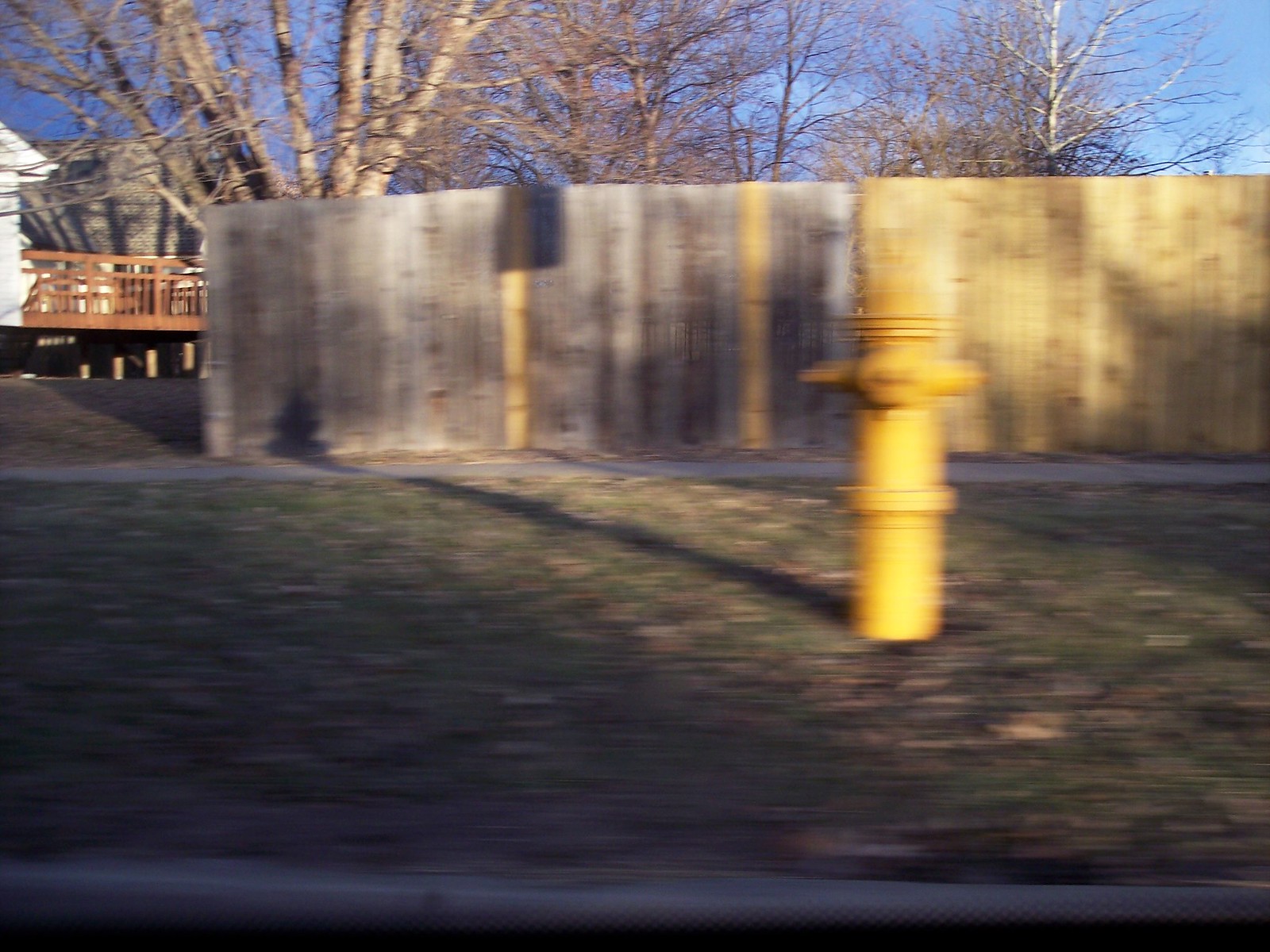This outdoor photograph, although very blurry and poorly focused, captures a winter scene dominated by leafless trees under a clear blue sky. In the background on the left-hand side, part of a white house with a gray roof and brown wood deck is visible. Surrounding this area is a wooden fence, basked in sunlight on the right side, stretching almost across the entire width of the image. There are brown and gray streaks on the fence, adding texture to the scene. In the middle right part of the image, there is a distinctive yellow fire hydrant standing amidst a patch of green grass mixed with scattered leaves. Adjacent to the hydrant, a concrete sidewalk runs in front of a concrete wall. The photograph appears as if captured in motion, contributing to its overall blur and giving the objects, particularly those in the bottom right corner, a sense of movement. The scene hints at a quiet neighborhood setting in the colder months.